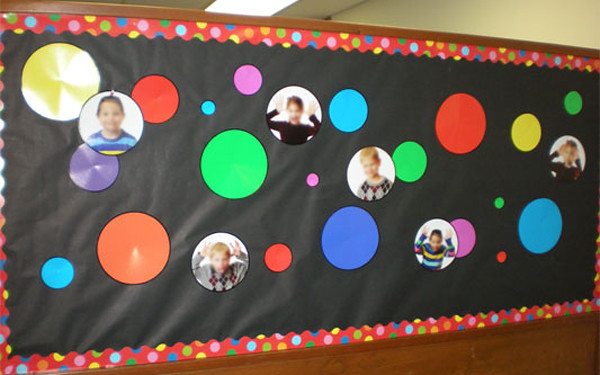The image showcases a colorful and somewhat blurry photo of a propped-up bulletin board, likely set in a classroom. The large, rectangular poster features a black background decorated with circles of various sizes and colors such as blue, orange, red, green, purple, and yellow. The border of the poster is a fun, party-balloon style, with a squiggly red border adorned with small, colorful circular elements in shades of light blue, green, orange, pink, and yellow. Scattered throughout the poster are six circular-framed photos of children making funny expressions, such as sticking their tongues out, positioned at the top left, bottom left, center, and right-hand side. The bulletin board itself is mounted on a wooden frame, and the top background of the image reveals part of the ceiling, emphasizing its classroom setting where children's artwork and photos are displayed.